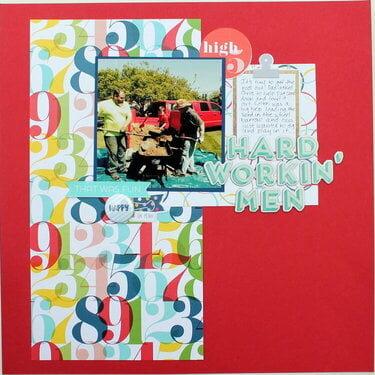This image appears to be a collage with a vibrant red background, featuring a distinct bubbly text in the forefront that reads "HARD WORKIN' MEN" in all caps, complete with a shadow effect to emphasize the lettering. To the left, a collection of multicolored numbers stand out, including a red 9, a blue 8, a light blue 6, a tan 4, a green 3, and a yellow 2. Hidden behind one of the primary images, there is a sticker-like element that says "HI" in white text on a pink background, accompanied by a number 5. Additionally, a circular button with the word "HAPPY" adds another layer to the collage.

The central image captures a scene involving a red truck with its rear open, suggesting it's ready for loading. In front of the truck, we see three individuals engaged in some sort of laborious activity. A hefty man is digging dirt out of a wheelbarrow situated on a green tarp, while a smaller, hat-wearing man and a younger child in a red t-shirt appear to assist him. These elements collectively indicate that this is likely a piece of handmade art or a designed card, illustrating the theme of hard-working men. The various components, including the multicolored numbers, text, and images, contribute to this intricate and colorful composition.